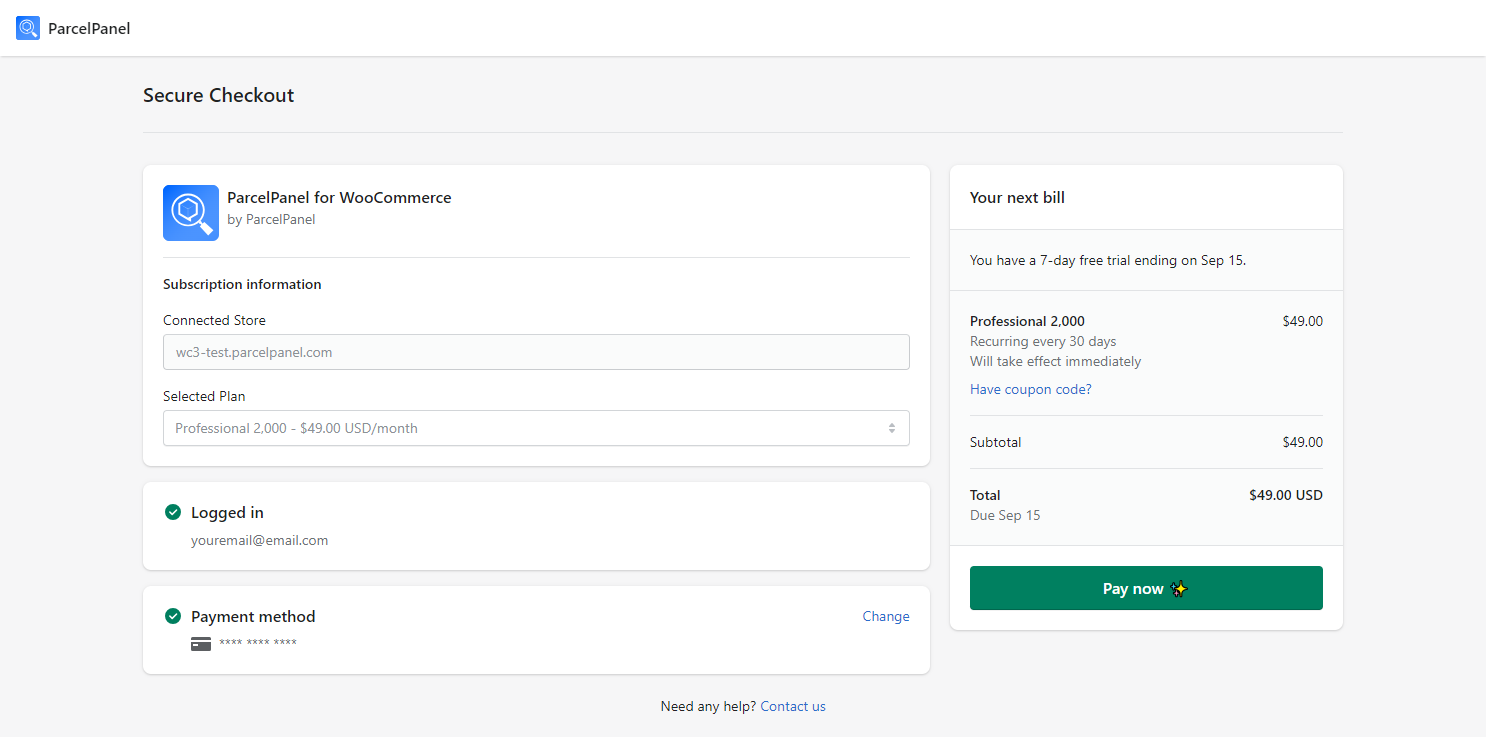The image displays the secure checkout page of the ParcelPanel website, specifically for the store "wc3-test.parcelpanel.com." The selected subscription plan is "Professional 2000," costing $49 USD per month. The page confirms the user's logged-in status with their email visibly displayed. Below this, the payment method is listed as a credit card, alongside a blue button allowing changes to this payment method. To the right, a detailed panel outlines the next bill, indicating the end of the 7-day free trial and the first charge of $49 on September 15. There's an option to apply a coupon for a discount. At the very bottom, a green "Pay Now" button with white text is prominently displayed.